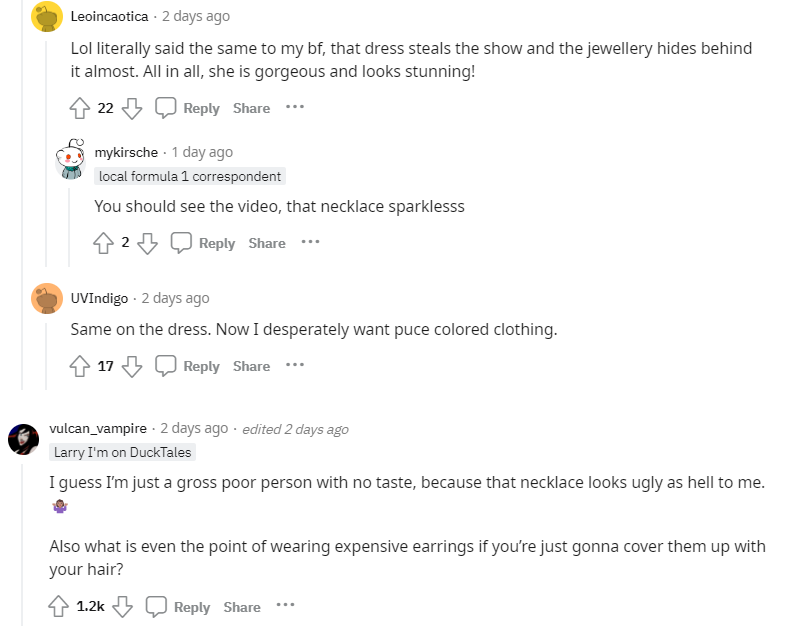Caption: 

A vibrant Reddit thread features a lively discussion revolving around fashion choices in an image. The top comment captures one user's admiration, stating: "Lol, literally said the same to my boyfriend. That dress steals the show and the jewelry hides behind it. All in all, she is gorgeous and looks stunning." Following this, another user chimes in: "She used to see the video; that necklace sparkles." 

A different user, UV ego, joins the conversation with: "Same on the dress! Now I desperately want to purchase colorful clothing." However, not all opinions are positive, as Vulcan Vampire interjects: "I guess I'm just a gross poor person with no taste because the necklace looks ugly as hell to me. Also, what is even the point of wearing expensive earrings if you're just going to cover them up with your hair?"

The thread is marked by typical Reddit interface elements including upvotes and user profile pictures. The screenshot is primarily black and white with hints of yellow and orange, highlighting the active user interactions.